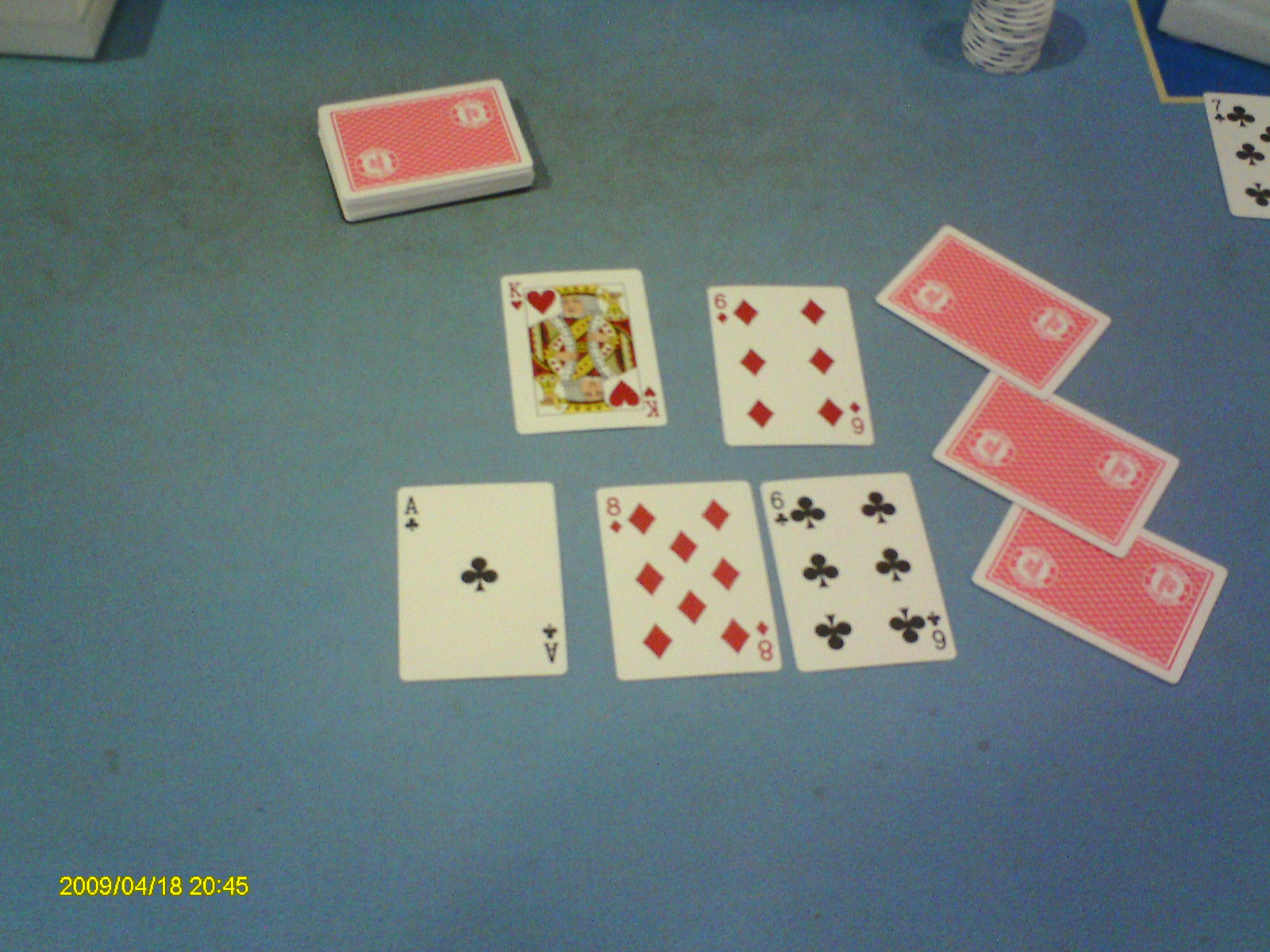The image features a gradient blue background that transitions from a greenish-blue hue at the top, sprinkled with tiny green dots, to a darker blue towards the right-hand side and bottom. In the upper left-hand corner, there is an indistinguishable white object casting a dark blue shadow. 

Prominently in the center is a stack of face-down cards, each white with a red rectangle and intricate red and white patterns. Scattered around are several face-up cards displaying various values: the King of Hearts at the top, to its right the Six of Diamonds, below that the Ace of Clubs, next to it the Eight of Diamonds, and next to that the Six of Clubs. Additionally, there are three more face-down cards identical to the initial stack.

In the upper right section, there's a small stack of poker chips, which are partially visible, and nearby, another distinctive chip with a yellow outline, blue inside, and a white interior. Below this chip is the Seven of Clubs.

In the bottom-left corner of the image, the date and time are marked in yellow text: "2009/04/18 20:45".